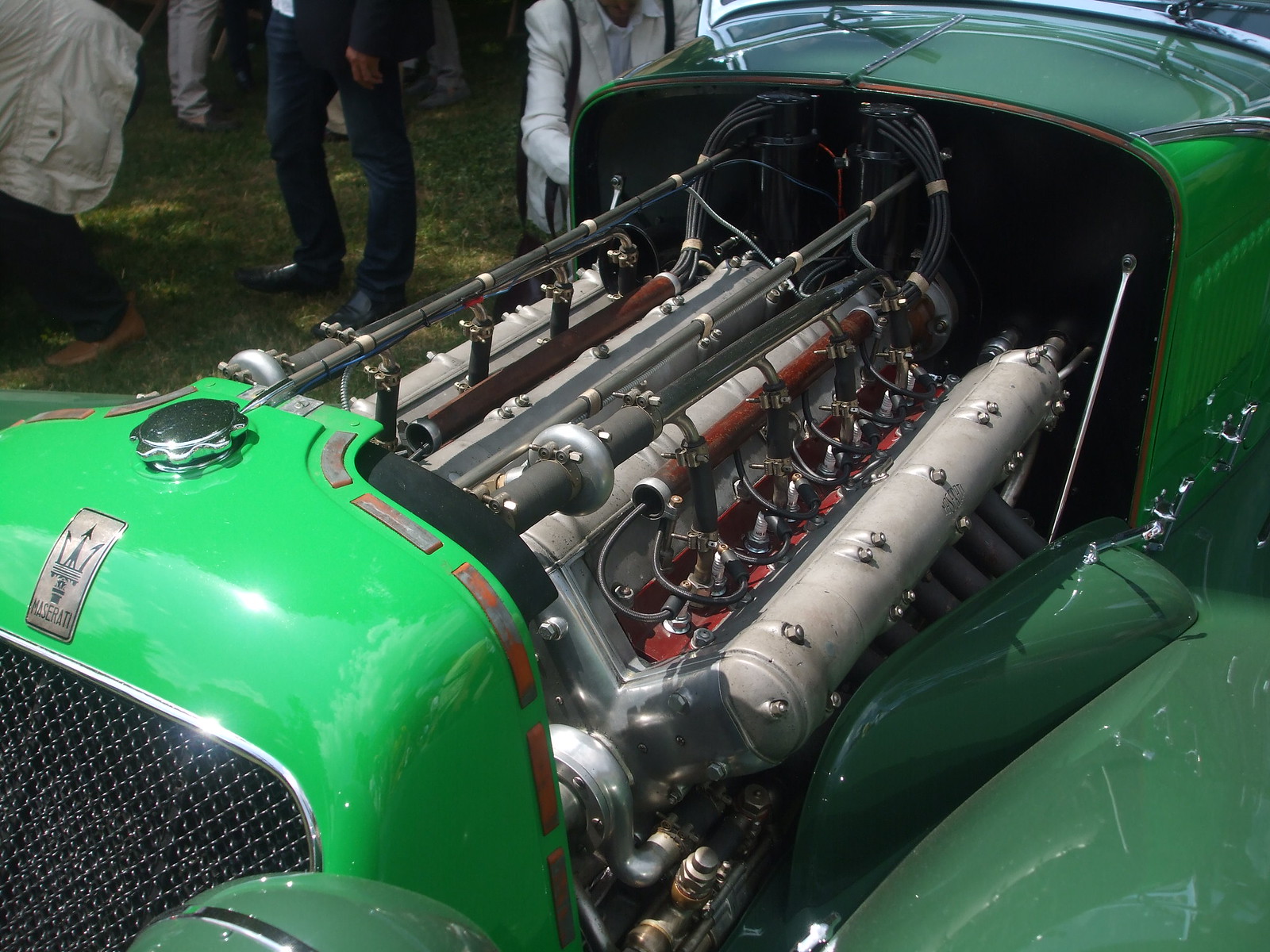This photograph captures a close-up of a meticulously maintained green hot rod at what appears to be an upscale antique car show. The focal point of the image is the car's large, exposed engine, which lacks a cover, showcasing its immaculate, spotless condition. The engine boasts significant components such as big headers and pipes connecting the oversized cylinders, accompanied by bundles of wires extending out to the core. The hot rod itself is a Maserati, as indicated by a visible badge on the front, featuring a curvaceous green frame with chrome elements that shine brightly under the sunny skies.

In the background, the scene reveals well-dressed individuals, standing on a grassy field, further emphasizing the high-class nature of the event. The photograph also captures a general ambiance of admiration, with multiple pairs of legs, suggesting the presence of spectators engrossed in the display. The overall setting suggests an outdoor venue filled with enthusiasts appreciating both the aesthetic and mechanical intricacies of this polished and well-preserved antique vehicle.